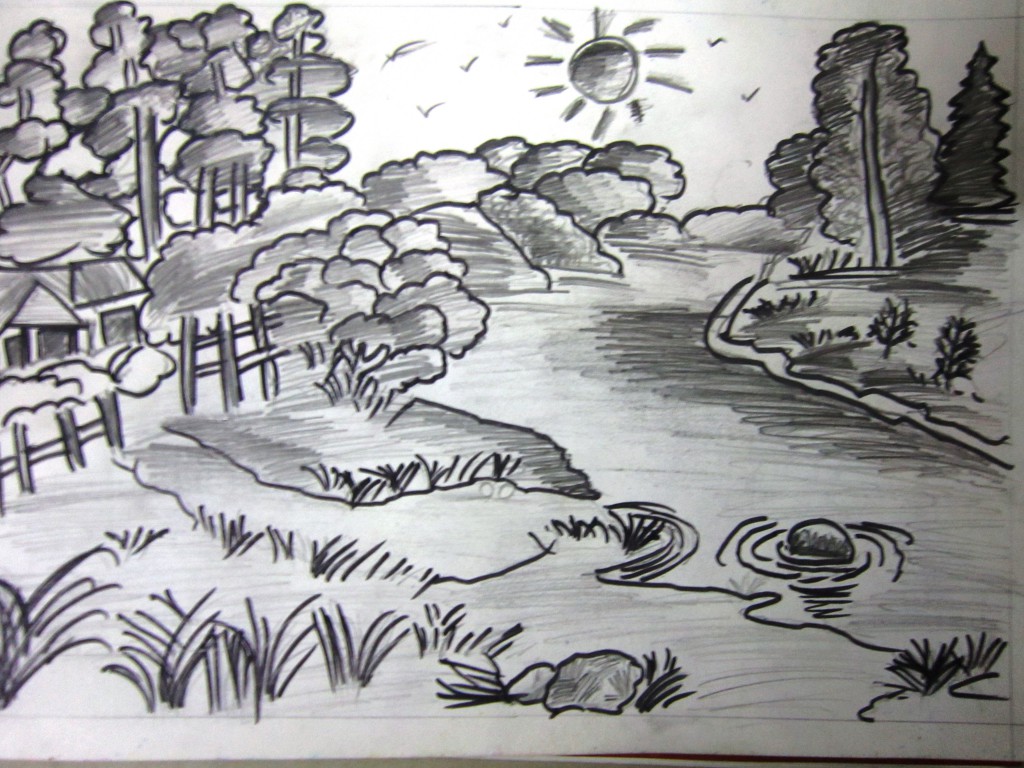This exquisite piece of pencil and marker artwork portrays a serene landscape that dominates the entire sheet of paper. At the heart of the composition flows a meandering river, flanked by a variety of shrubs and punctuated by clusters of taller trees in the background. The sun, positioned at the center top of the drawing, radiates light with distinct rays and is accompanied by several V-shaped birds soaring through the sky.

In the foreground, meticulously rendered details include an array of rocks and tall grasses, contributing to the textural depth of the scene. A charming cottage sits on the left bank of the river, surrounded by a quaint fence that adds to the idyllic setting. Dominating the right side of the river, a mixture of tall pine trees and younger ones sprouting up create a lush, varied forest.

Executed entirely in shades of gray and black on pristine white paper, this monochromatic artwork captures the tranquil beauty of nature with remarkable detail and contrast.